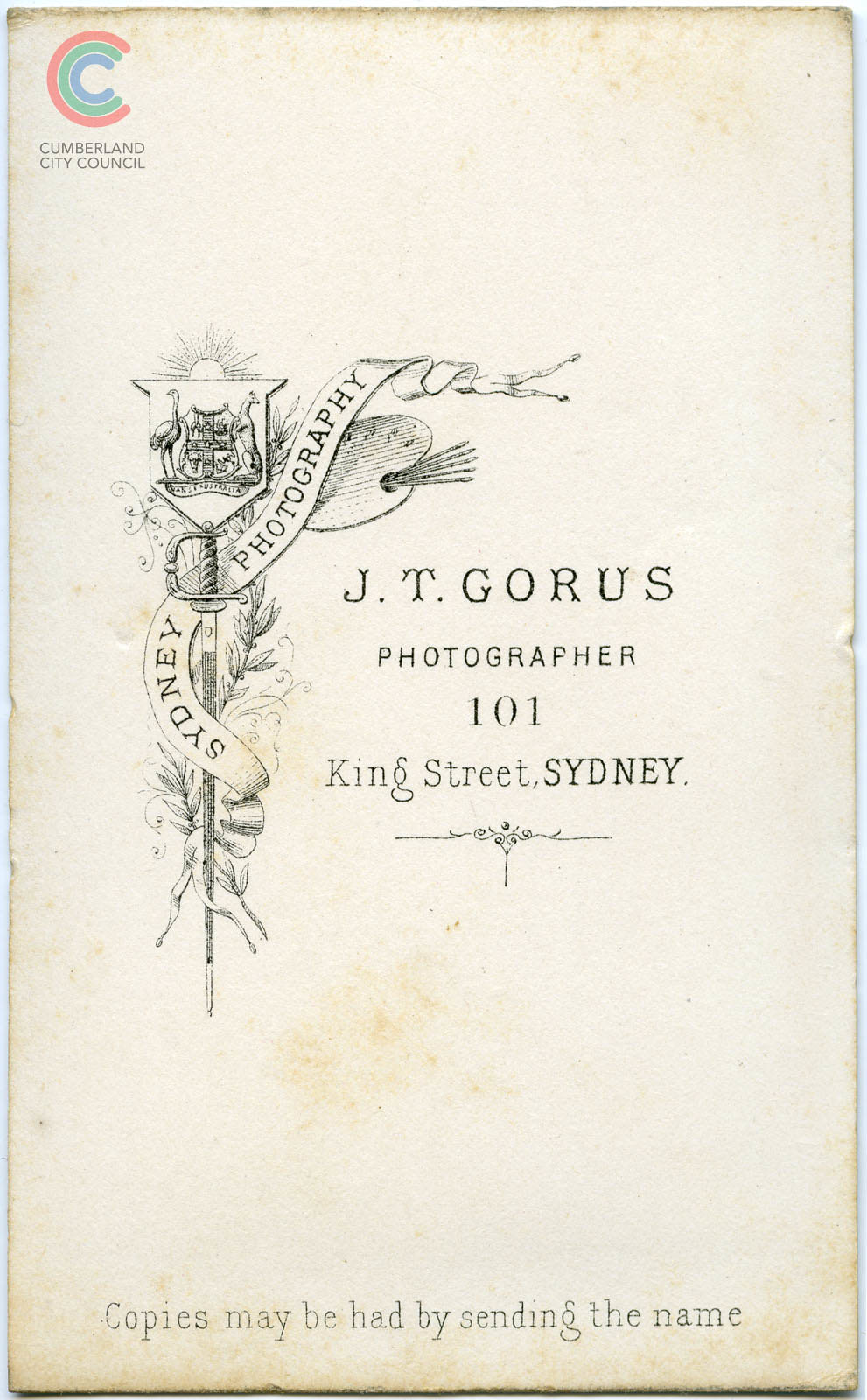This image depicts an advertisement from an old, scanned book cover belonging to photographer J.T. Goris, whose studio is located at 101 King Street, Sydney. The paper has aged, displaying a beige background with brownish and yellowish dirt marks, particularly along the bottom and in the corners. The top left corner features the Cumberland City Council insignia, a logo comprising concentric 'C' shapes in blue, green, and light red, mimicking the appearance of a sea. Centrally, the cover showcases a detailed black and white drawing of a shield adorned with the figure of an ostrich and a kangaroo, encircled by leaves. A ribbon inscribed with "Sydney Photography" wraps around a pole resembling a sword. Below the drawing, in bold black text, the name J.T. Goris, photographer, is prominently displayed. At the bottom of the cover, it reads, "Copies may be had by sending the name."